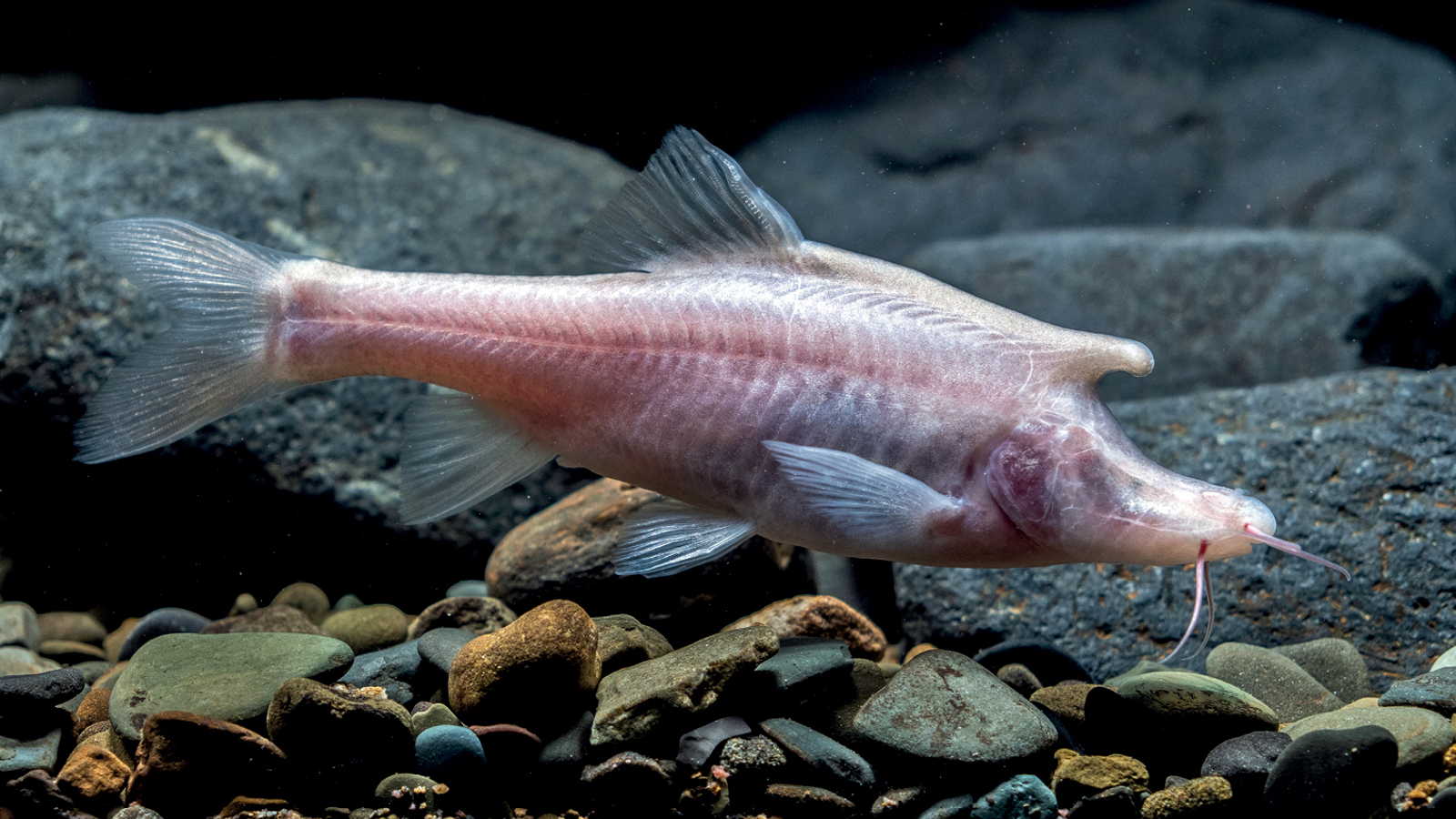The image is a detailed color photograph of a cynocyclocheilus longicornis, a rare fish primarily found in the dark waters of southwest China. This small fish is characterized by its pink, semi-transparent body and striking silver-gray fins. Notably, it features a long, needle-like snout adorned with four prominent whiskers. Swimming towards the right side of the image, the fish is depicted in a clear aquarium setting. The bottom of the tank is lined with an assortment of small brown and gray pebbles, while larger dark gray rocks create a backdrop. The photograph is taken underwater, emphasizing the clear water and semi-blurred background. The overall setting and style of the image is indoors and aquatic, showcasing photographic realism in wildlife and underwater photography.